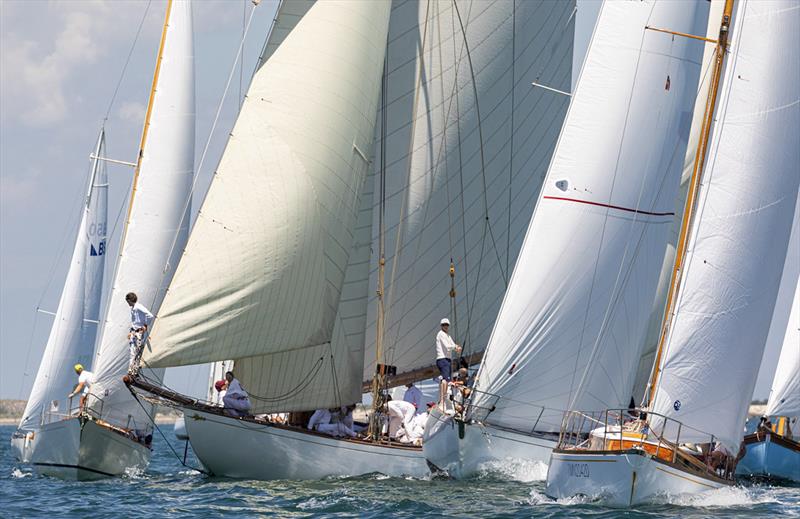In bright sunlight, a fleet of luxury sailboats, five clearly visible and possibly more in the distance, are navigating a serene body of water, likely the ocean or a bay. These sleek vessels, predominantly white with towering sails that vary from pristine white to off-white with minimal stripe details, appear to be engaged in a close-knit race or regatta. They are tightly clustered together, their hulls almost touching, which seems unusual. Each boat has men in white attire, with several standing prominently at the very front, gripping the railing or the mast. The hint of slight waves and the arrangement of the boats suggest they're in motion, sailing in unison towards the observer. Notably, one sailboat on the right has a blue hull, adding a splash of color to the otherwise uniformly white scene.